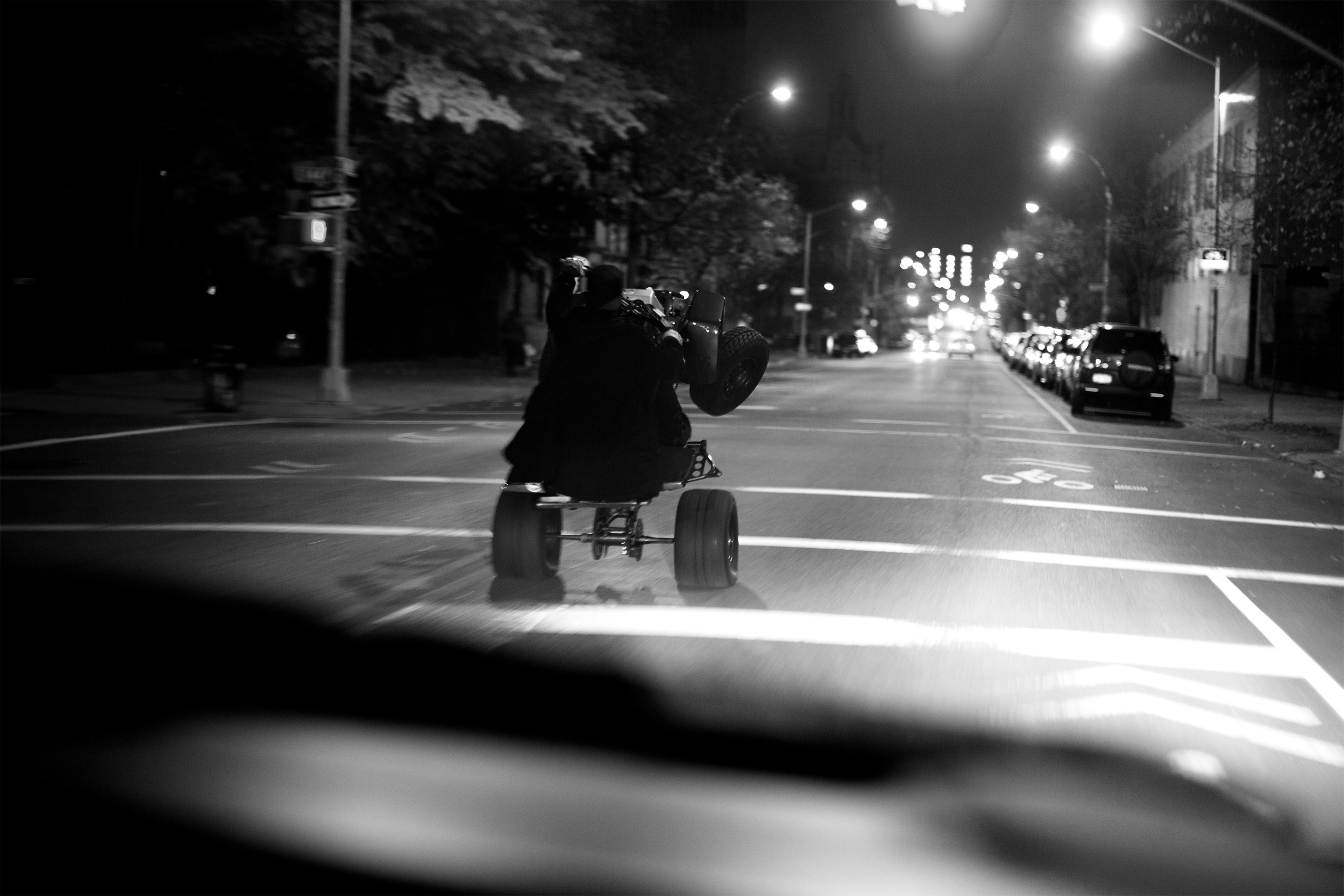This atmospheric black and white nighttime photo captures the view from a car following closely behind a person performing a stunt on an ATV. The rider, dressed in a long, dark coat and hat, is balancing the vehicle on its two rear wheels. The scene unfolds at a straight, four-way intersection illuminated by streetlights and marked with crosswalks. Trees line the left side of the street, while several cars are parallel parked along the right. The background features tall buildings reminiscent of a bustling New York City street, adding depth to the urban landscape.